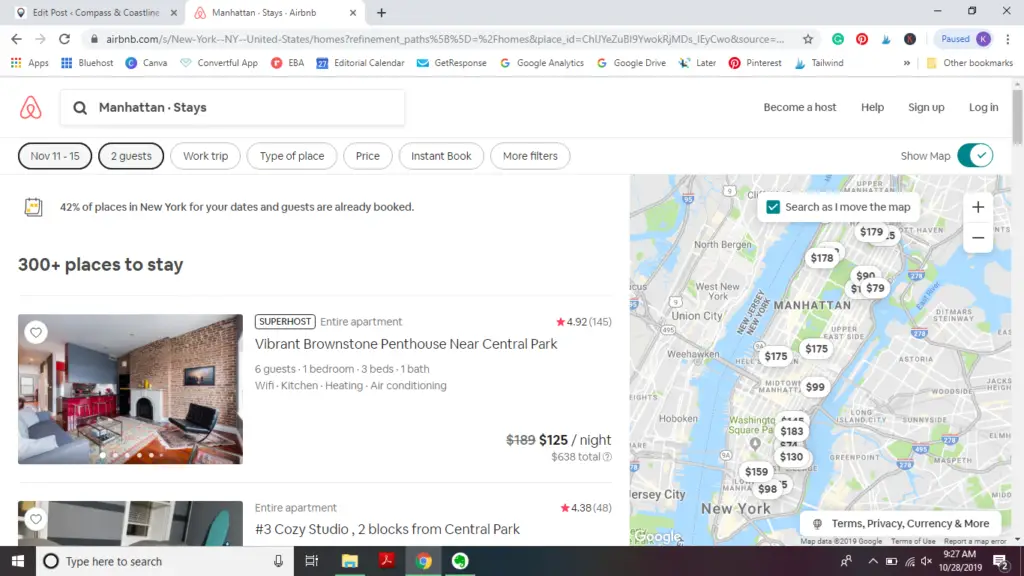Screenshot of a Manhattan Stays Search on Airbnb

This image is a screenshot of a computer monitor displaying a web page with Airbnb search results for accommodations in Manhattan. The screenshot, captured from a Google Chrome browser window, shows two tabs: the active tab is titled "Manhattan stays Airbnb," and the other, inactive tab mentions “Eastport.” The browser's URL bar is visible, indicating the search query.

The Airbnb search page details various options and filters, reflecting a search for stays in Manhattan for two guests from November 11th to 15th. The user has selected the “Show map” feature, which displays accommodations on a Manhattan map to the right. Above the search results, there are options for users to become a host, seek help, sign up, or log in. Additional filter categories like “Work trip,” “Type of place,” “Price,” “Instant book,” and “More filters” remain unselected.

A prominent notification on the page indicates that 42% of places in New York for the selected dates are already booked, yet over 300 places are still available. The top search result illustrates a “Vibrant Brownstone Penthouse near Central Park” with a 4.92 rating based on 145 reviews and a nightly price of $125, recently reduced from $189. The listing specifies it is for the entire apartment. Another result listed is a “Cozy Studio, two blocks from Central Park” with a 4.38 rating.

The map of Manhattan visible on the right side of the screen shows various prices for accommodations across Manhattan, though it does not highlight the specific listings mentioned. 

At the bottom of the screen, the Windows taskbar is discernible, showing icons for File Explorer, Adobe, Chrome, and a few other programs. The far-right corner of the taskbar displays system indicators for laptop battery, Wi-Fi, volume, time, and date.